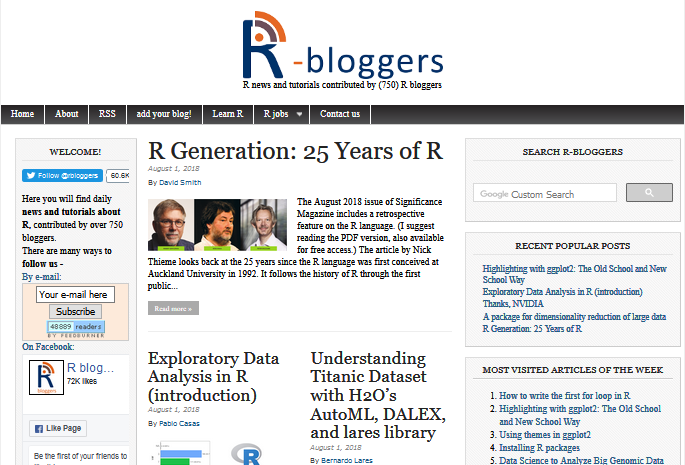The image showcases the R-bloggers website prominently centered in the frame. At the top, the site's name is displayed with "R" in a significantly larger and capitalized font, serving as the logo to the left of the word "bloggers," which is in lowercase letters. Below the site name, a tagline in smaller font reads, "R-bloggers: News and tutorials contributed by 750 R bloggers."

Directly beneath the tagline, there is a horizontal navigation menu bar stretching from the left to the right side of the screen. The menu includes links labeled "Home," "About," "RSS," "Add Your Blog," "Learn R," "R Jobs," and "Contact Us."

The main content area of the website is divided into three sections. On the left, there is a vertical welcome section introducing the site and its purpose. Central to the layout is a prominent article titled "R Generations: 25 Years of R," accompanied by an image or graphic, highlighting a significant milestone for the R programming community. Below this article, additional blog posts and news articles are arranged, continuing to provide valuable updates and insights.